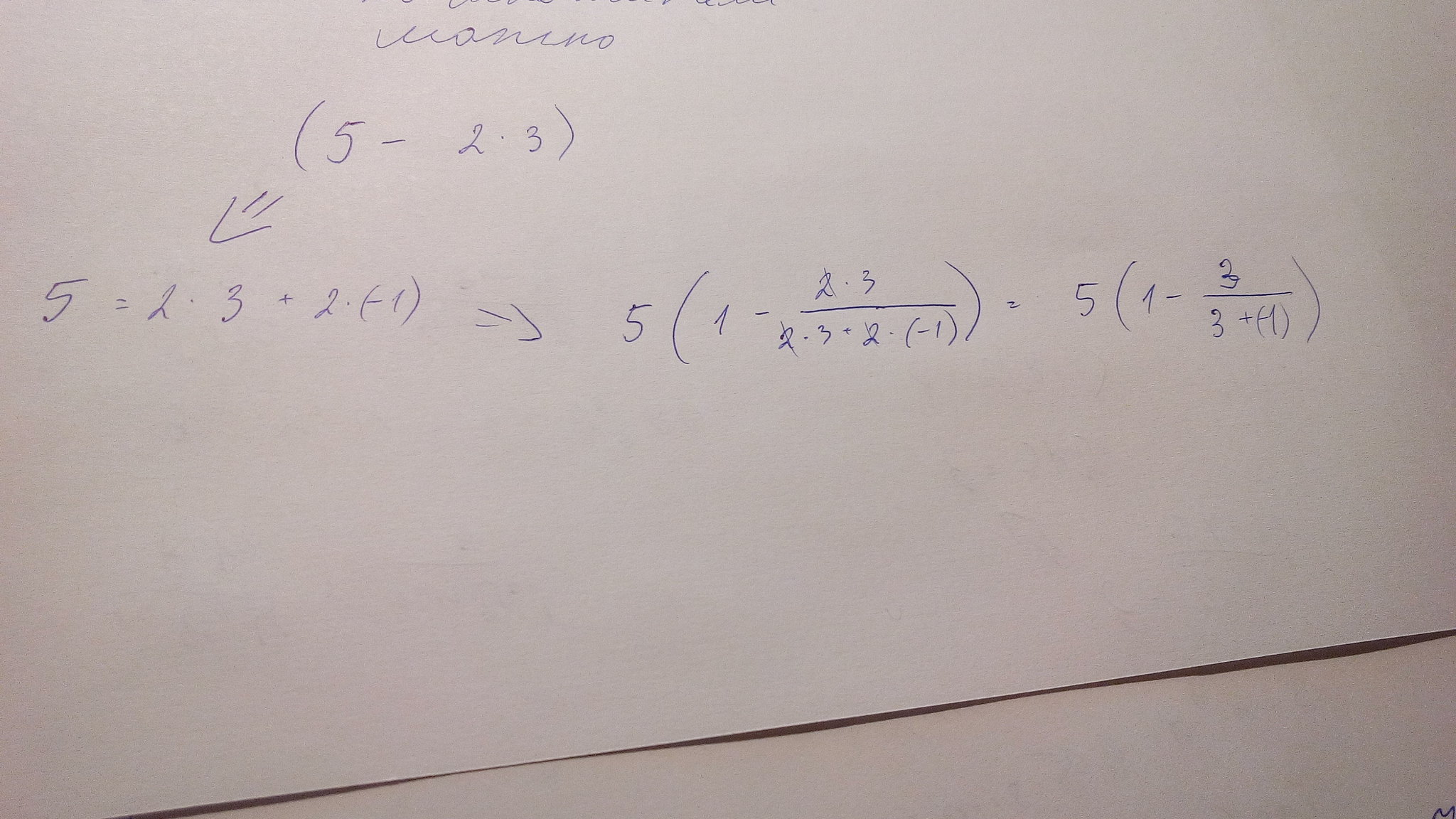This photo captures a complex mathematical equation written on a chalkboard. The equation in question is: \(5 = 2 \times 3 + 2 \times (-1) \Rightarrow 5 \times (1 - 2 \times \frac{3}{2}) \times (3 \times 2 \times -1)\). In an effort to simplify the problem, the equation evolves to \(5 \times (1 - \frac{3}{2}) \times (3 + (-1))\). The overall scene suggests a moment of deep concentration and intellectual pursuit, emphasizing the meticulous steps involved in solving advanced math problems. The chalkboard is filled with various mathematical operations displayed in layers, offering a glimpse into the problem-solving process.